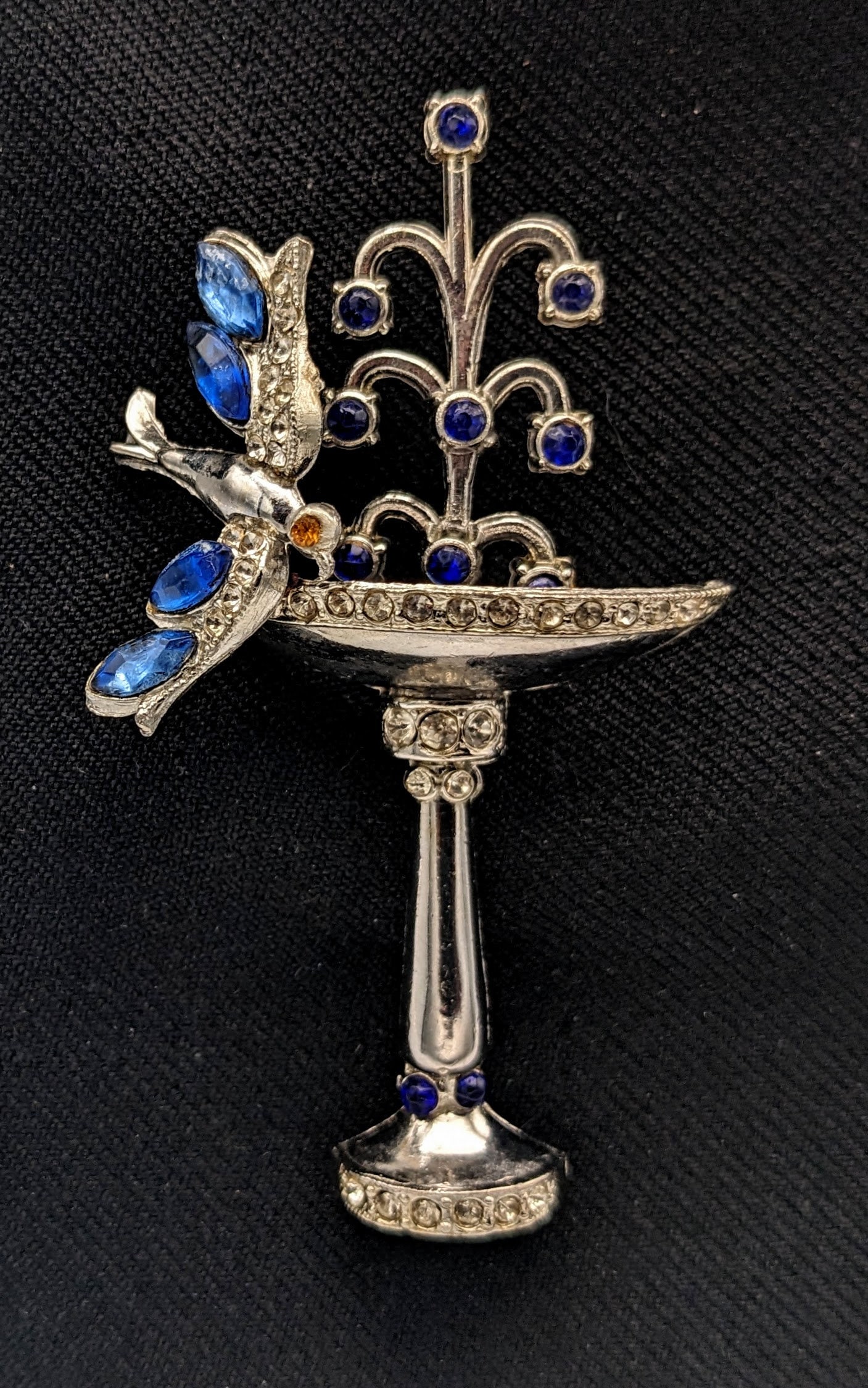This close-up photograph features an intricately detailed silver brooch pin set against a black fabric backdrop. The brooch, crafted from a shiny, metallic silver material, depicts a birdbath atop a pedestal, elegantly designed to resemble an ornate fountain. The water jets, represented by silver curls, are adorned with deep blue, almost purplish gemstones. Among these, the birdbath forms the central motif, leading up to the fountain's water arcs, each terminating in a glistening blue gem. 

On the left side of the brooch sits a beautifully crafted bird, its wings encrusted with multiple blue gemstones, and sporting a striking orange gem for its eye. The bird's metallic feathers, tail, and wings reflect the same shiny silver finish. Additional white or clear gemstones embellish the piece, adding to the brooch's dazzling appearance. The absence of any text or extra elements in the photo highlights the elegance and detailed craftsmanship of the jewelry.